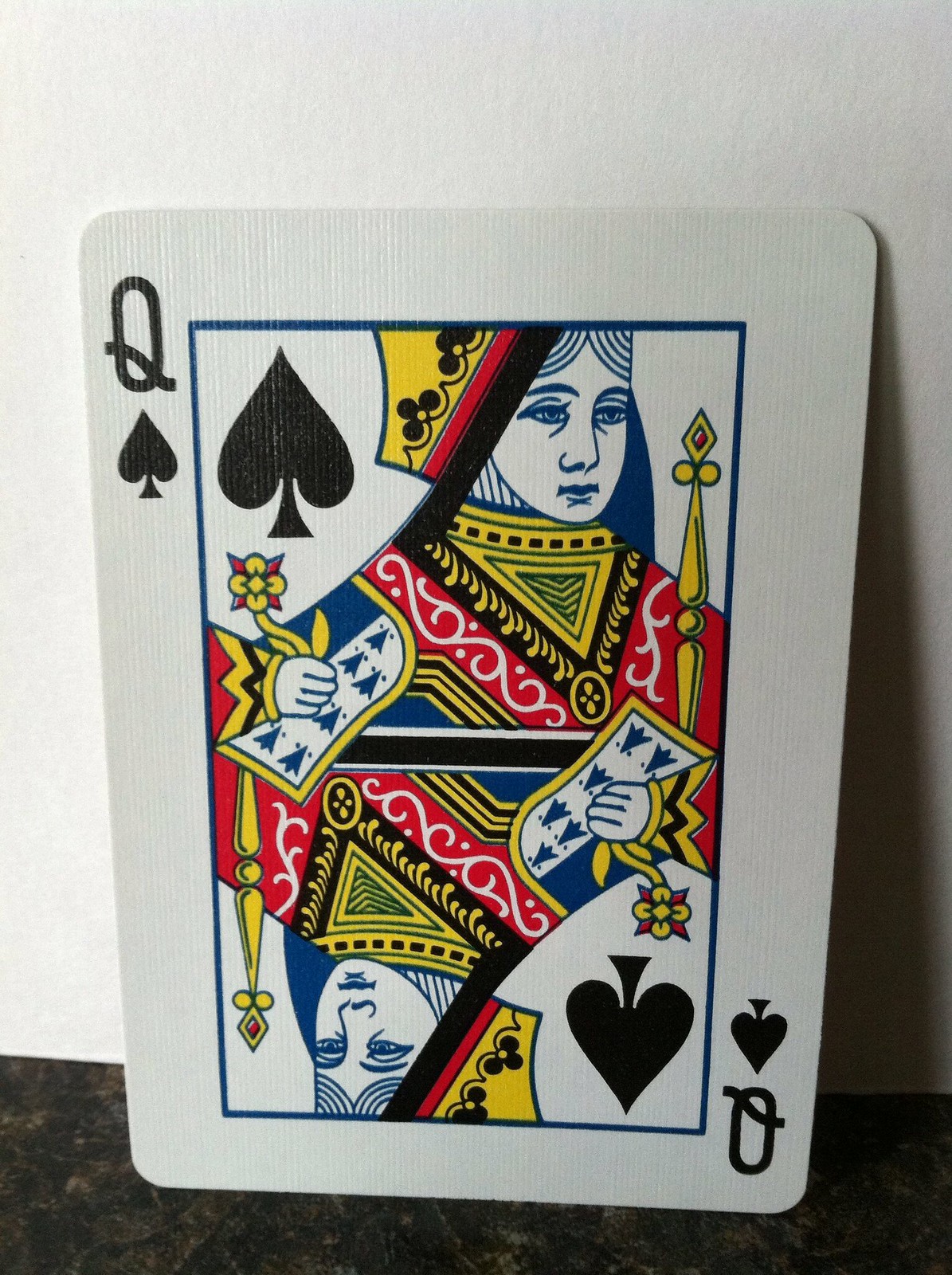This close-up image features the Queen of Spades playing card prominently displayed on a black counter. The card is tilted against the wall, showcasing its intricate design. The background contrasts starkly with the white card, highlighting its detailed features. Emblazoned in both the upper left and lower right corners are the "Q" and spade symbols, traditional markers of the card. 

The center of the card depicts the Queen herself, adorned with a yellow crown and clothed in a red dress accented by a striking blue collar. Her expression is poised and regal, and in one hand, she clutches an ornate, unidentified object. The mirrored image of the Queen appears upside down beneath the main depiction, maintaining the card’s symmetrical design. 

The color palette of the card is a blend of crisp whites, deep blacks, muted grays, vibrant reds, yellows, and a touch of dark blue. Despite being a commonplace playing card, the picture emphasizes its classic and timeless design through focused detail and contrasting colors.